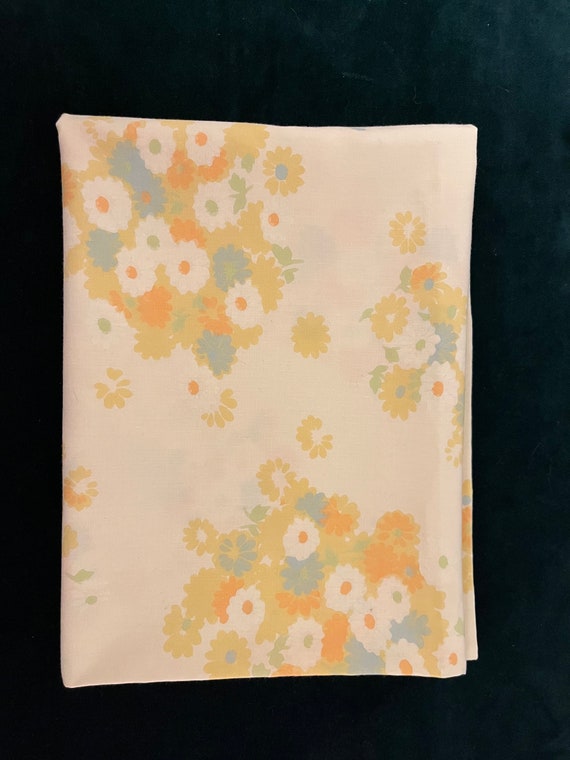This is a photograph of a neatly folded piece of linen, resting on a nearly black background. The linen, possibly a sheet or tablecloth, is an off-white or cream color and features a detailed floral design. This design consists of various daisy-like flowers, each with 12 petals radiating from a solid center. The flowers are depicted in an array of colors—yellow, orange, blue, and green—some using negative space to appear white. The centers of the flowers vary in color, including green, orange, blue, and yellow. The floral patterns are arranged in clustered formations: a large cluster near the bottom right, another near the upper left, and a smaller cluster midway up the right side, along with several single flowers scattered throughout. The pastel and matted hues of the flowers contribute to the linen's overall attractive and artistic appearance.